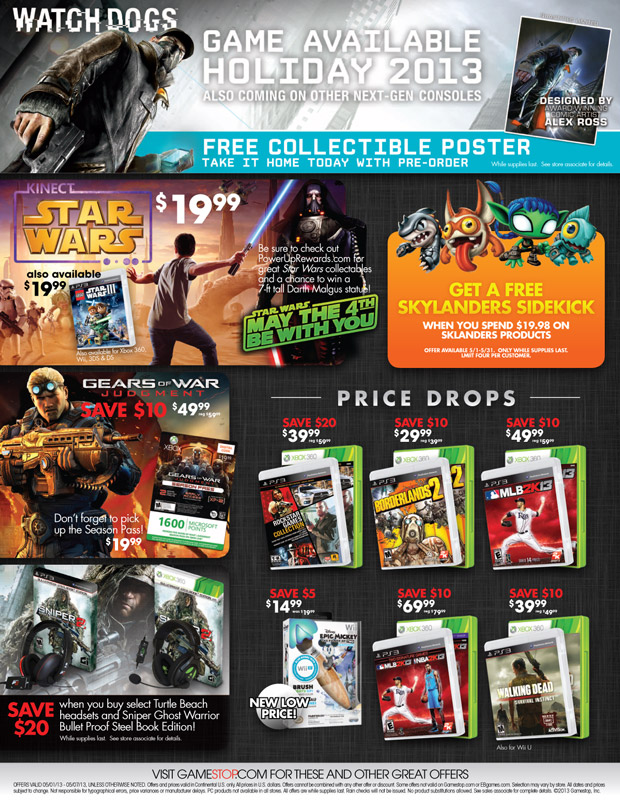This is an intricate promotional webpage advertising various video games and related merchandise. At the top of the page, there's a prominent banner for "Watch Dogs," featuring a foreboding character whose face is obscured by a hat, viewed from a low angle. The text highlights that the game will be available during the holiday season of 2013, and mentions, "Designed by Alex Ross," accompanied by an image that likely depicts the same enigmatic character. Additionally, there’s an enticing offer for a free collectible poster with a pre-order, alongside a note that the game will be released on other next-generation consoles.

To the right, another highlighted promotion showcases "Kinect Star Wars," with the tagline "May the 4th Be With You." This section includes visually engaging images from the movie or video game, noting that the product is available for $19.99. Furthermore, a special offer is detailed: customers can receive a free Skylander Sidekick by spending $19.98 on Skylander products, presented in an orange box with characters peeking over its edge.

Continuing the promotional content, there's a segment titled "Gears for War," offering significant savings of $10, bringing the price down to $49.89. This section includes a display of six games, each highlighting potential savings and corresponding prices, appealing to budget-conscious gamers.

At the bottom, there's a special promotion that offers $20 savings when purchasing select Turtle Beach headsets and Sniper Ghost Warrior Bulletproof Steelbook Editions, accompanied by an illustrative image of these products. The caption encourages users to visit GameStop.com for these deals and other exciting offers, concluding the ad-rich webpage with a call to action.